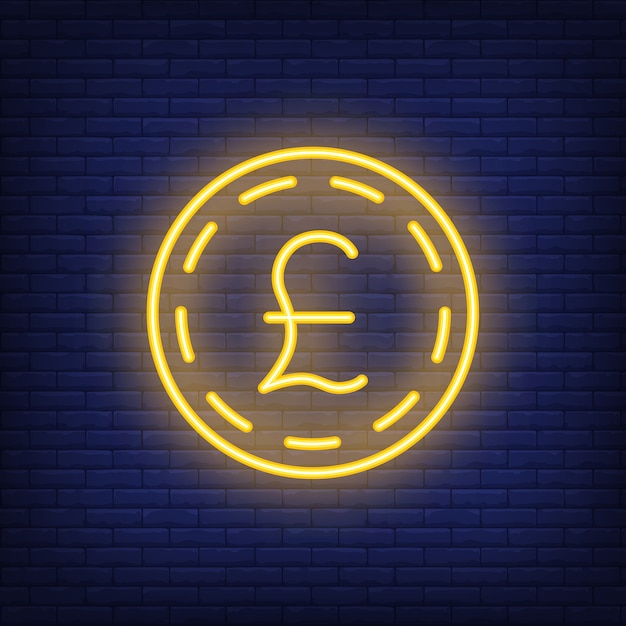The image portrays a perfectly square photograph with a strikingly detailed scene. It features a dark purple brick wall that transitions from a nearly black gradient in the corners to a lighter, more illuminated center due to a neon sign. The neon sign itself consists of a brilliantly lit yellow circle with a smaller, dashed yellow circle nestled inside. At the very center of this composition is a glowing yellow symbol resembling the British pound sign (£), characterized by a hook-like figure with a curly leg and a cross stroke. The neon light casts a yellowish hue onto the surrounding bricks, further accentuating the vividness of the symbol and circles against the dark, textured background.